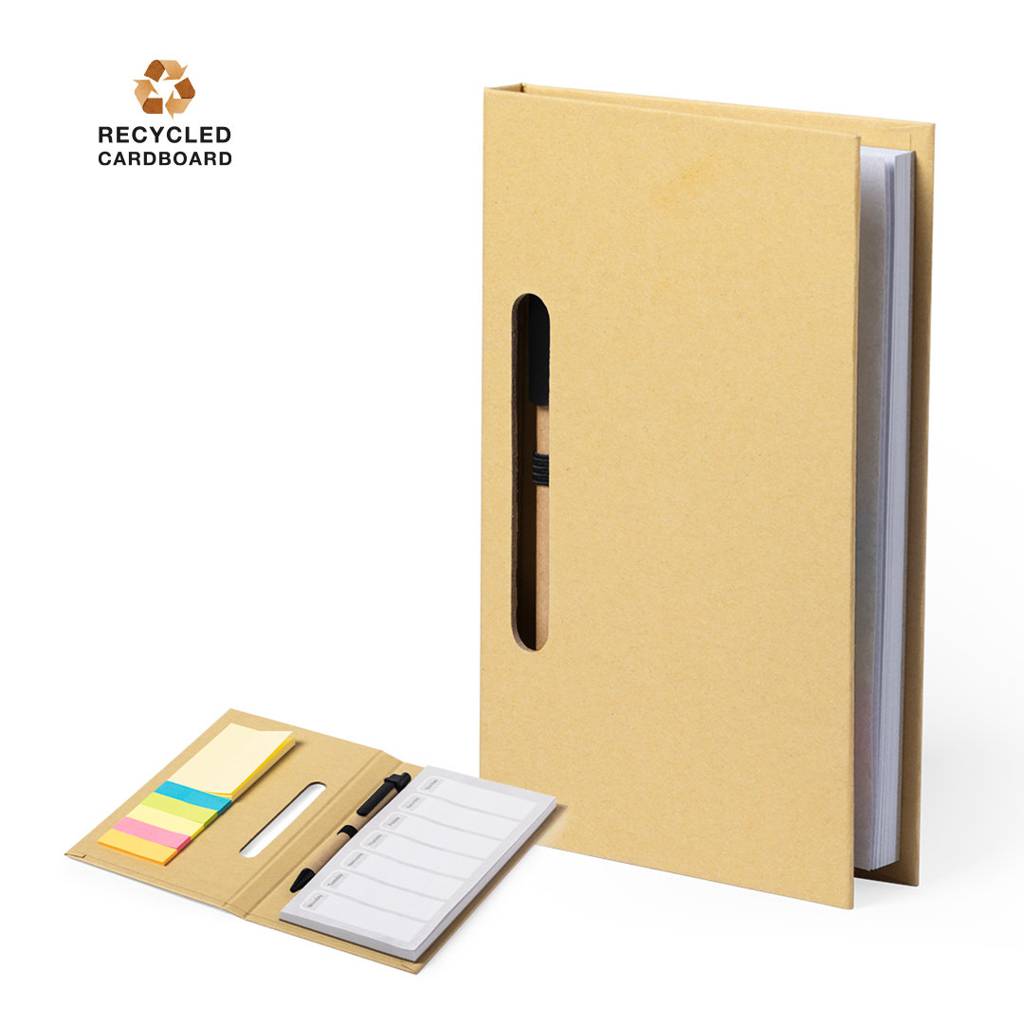The photograph depicts an advertisement for a stationery set crafted from recycled cardboard. Set against a stark white background, the image features a deep cream-colored journal with a hardcover standing upright at a slight angle. The top left corner of the image prominently displays a recycling logo in a cardboard brown hue, accompanied by the text "recycled cardboard" in black. 

The journal reveals white pages inside, although it is uncertain if they are lined. There's a clear slot on the front cover designed to hold a pen, which is also included and matches the journal's cream color with black trimmings. To the left of the standing journal, there's a smaller version opened up, showcasing lined paper inside, sections for daily documentation, and an array of sticky notes in yellow, blue, and pink attached to the left cover. The cohesive design of the stationery set, complemented by a matching pen, underscores its eco-friendly and practical appeal.